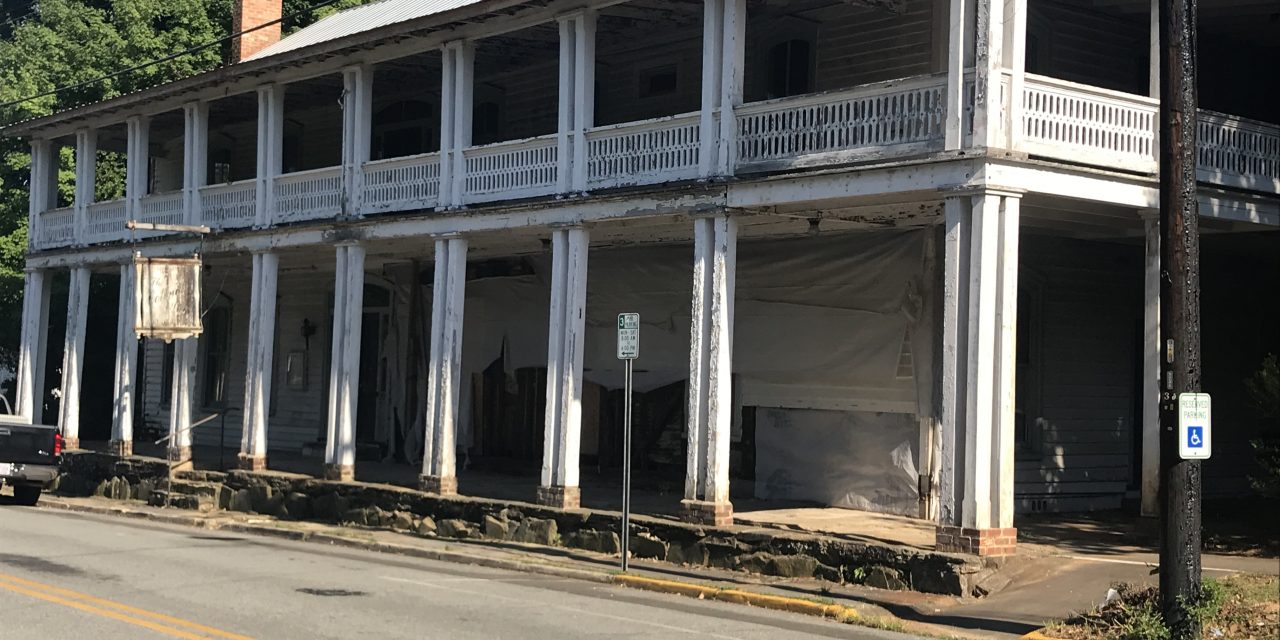The image captures a dilapidated, abandoned two-story building, likely a former inn, characterized by ten white, wooden columns extending from the base to the second-story balcony. The columns, painted white and equidistantly spaced, appear weathered with visible scratches. The building's facade is lined with deteriorating white siding, and the bottom porch is draped with dirty, white sheets. A set of steps leads up to the entrance. In the foreground, an asphalt street features a three-hour parking sign near the curb, and a black truck is parked or driving by. To the right stands a burned telephone pole adorned with a handicap parking placard. In the top left corner of the image, lush green trees are visible, adding a stark contrast to the rundown state of the building. A damaged sign hangs precariously from the upper left side of the structure, further emphasizing the abandonment and decay.